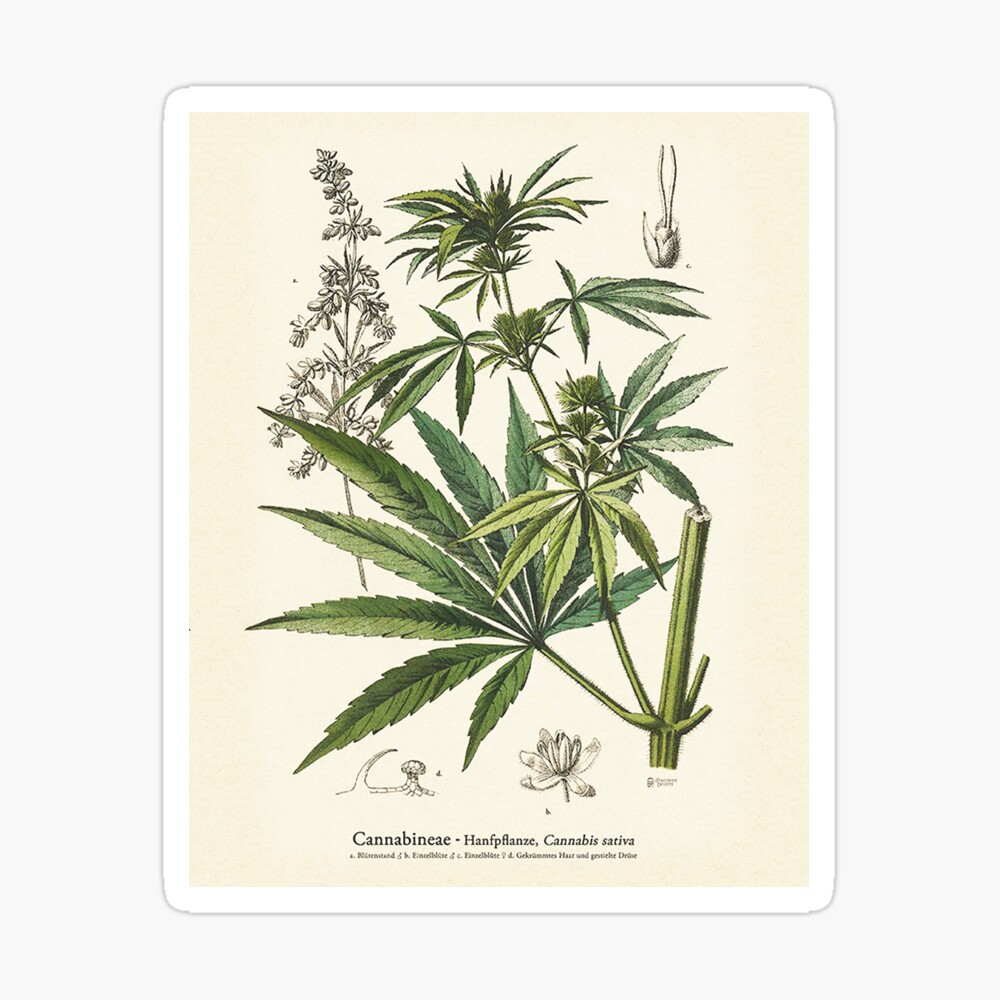This detailed illustration showcases various stages of a cannabis plant, scientifically named Cannabis sativa, with botanical precision. At the bottom of the image, the text "cannabinae" is prominently displayed in black, accompanied by the Latin name “Cannabis sativa.” The central drawing vividly portrays the mature cannabis plant with its green fan-shaped leaves, each leaf consisting of long, slender leaflets, typically eight in number. Stems branching out from the main stem are also meticulously detailed in green.

Surrounding the main colored illustration, other black-and-white sketches provide additional insights into the plant’s development. In the top right corner, an early growth stage is depicted, where tiny sprouts emerge from a seed, resembling delicate antennae. On the left side, there's a mid-growth sketch, illustrating the plant as it progresses through its growth cycle. Another close-up drawing zooms in on the multi-leaf structure of the cannabis leaf. Additionally, a detailed sketch of a bud is included on the upper right, and a cross-sectional view of the stem reveals the interior texture, shown in a tan color.

Overall, the illustration merges detailed visual renderings with scientific annotations, effectively conveying the cannabis plant’s anatomy and stages of growth.